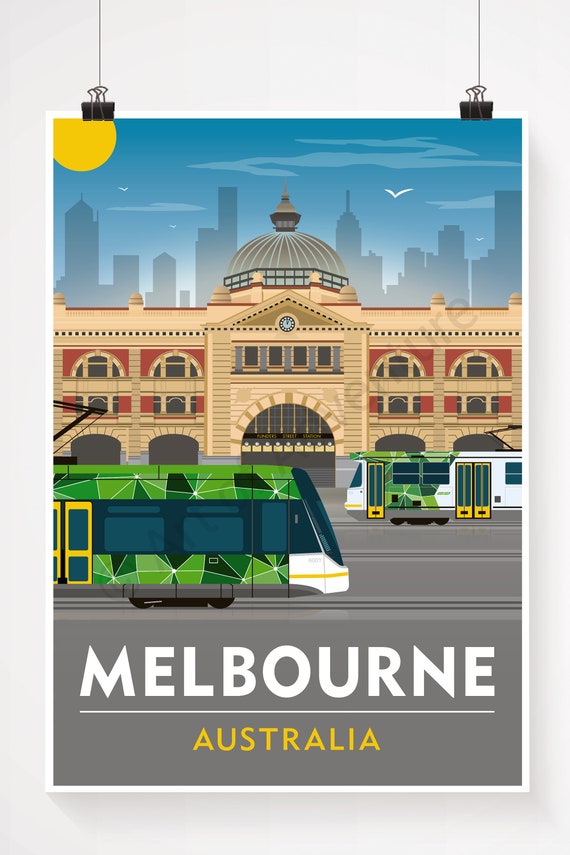This digitally painted infographic-style poster for Melbourne, Australia, features bold watercolor-like colors and intricate details. At the bottom, in all-capital white letters, it reads "MELBOURNE," with "AUSTRALIA" in smaller, capitalized yellow letters underneath. The foreground showcases two light rail trains: the nearest one is predominantly green with white accents, while the one behind it is mostly white with green and yellow detailing. These electric streetcars traverse light rail tracks set against a gray asphalt street.

Central to the image is a grand, vintage-style train station adorned with a dome, red accents, and numerous windows and arches, suggesting historical architecture. Above the station's intricate facade, though the text on it is too small to read, the cityscape of Melbourne unfurls into the background with a skyline rendered in gray outlines. Completing the scene, a blue sky with wispy clouds, a white bird, and the sun positioned in the top left corner create a vibrant and lively depiction of the city. This polished, minimalist computer graphic painting is hung on a white wall using two binder clips and black strings, adding a modern touch to its presentation.